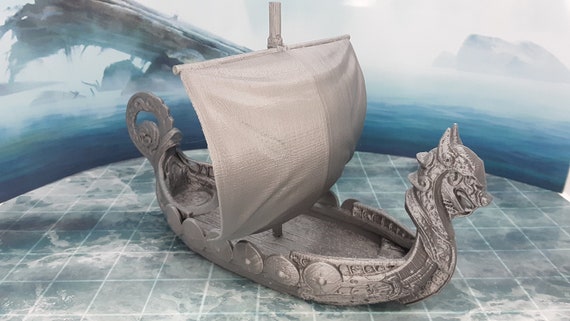The photograph showcases a meticulously 3D-printed Viking ship, situated at the center of a rectangular image with dimensions where the top and bottom sides are twice as long as the left and right. The Viking ship, rendered entirely in a single, unsanded gray, is adorned with the characteristic ridges from the 3D printing process, giving it a rough texture. The ship features a dragon-themed design, with a fierce dragon's head at the bow and a curling dragon's tail at the stern. Along either side of the ship, round shields are aligned along the railing. The ship's sail, also gray and square-shaped, appears to be billowing forward, adding to the dynamic nature of the scene.

Supporting the Viking vessel is a tile-like grid panel underneath, designed to mimic an icy, stormy ocean. The background of the photograph is a curved display, depicting a vast icy landscape with water and rocks, enhancing the overall thematic representation. The ship is slightly angled, with the bow pointing closer to the viewer on the right side and the stern farther back on the left. This silver-colored ship model, imbued with historical and mythical elements, stands as the focal point amidst a setting that suggests a cold, turbulent sea voyage.